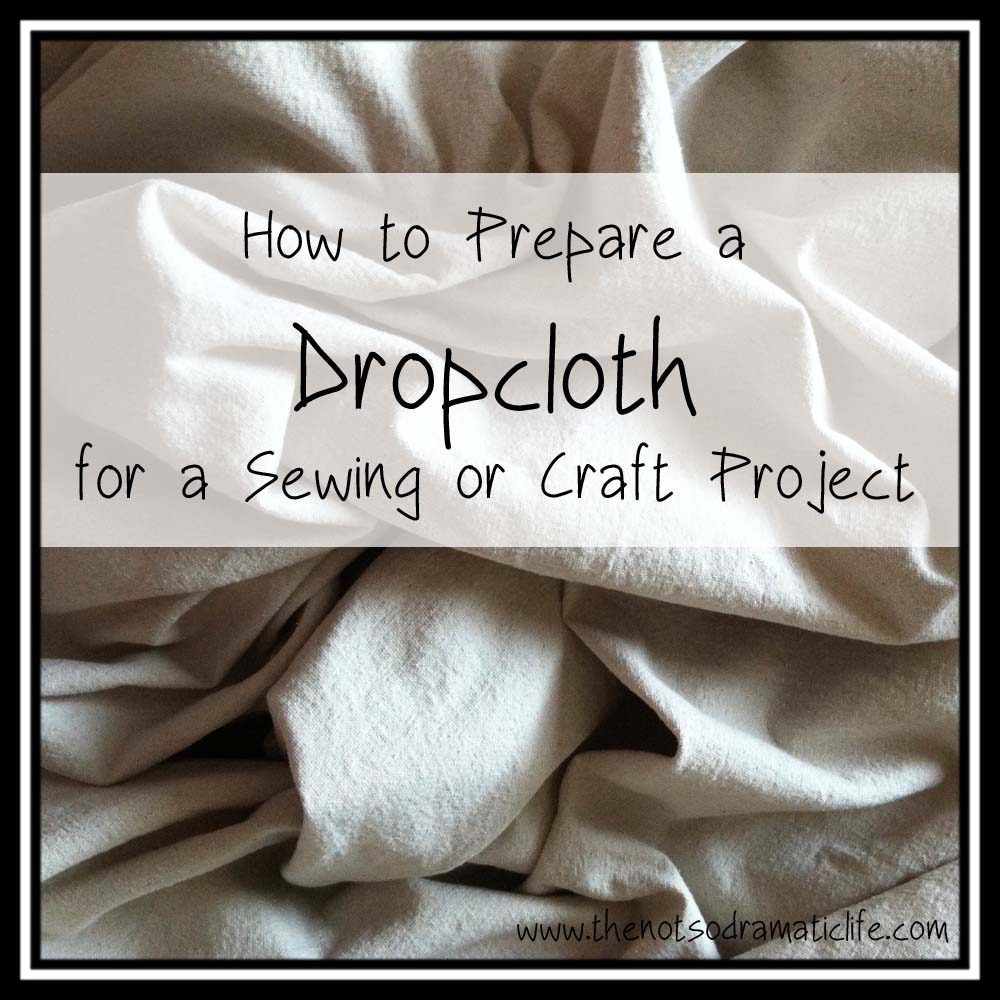The image is a title card featuring a black frame, with an inner white border followed by another black border. Inside the innermost black frame, there is a photograph of a heap of white or cream-colored linens, casually piled up rather than neatly folded, showcasing their texture and folds. Over the linens, there is a partially translucent, faded white banner with black text that reads, "How to prepare a drop cloth for a sewing or craft project." In the bottom right corner of the image, the website URL "www.TheNotSoDramaticLife.com" is displayed in black text.